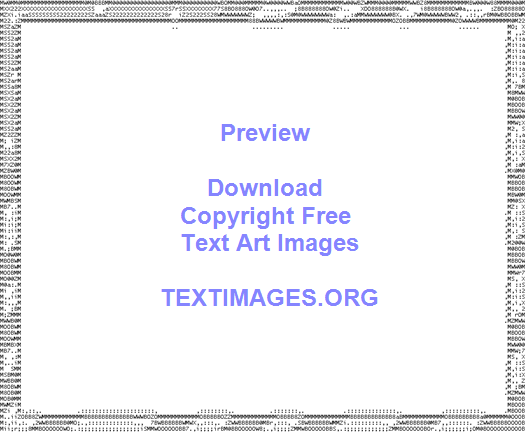The image depicts a digital artwork that resembles a picture frame created entirely from keyboard characters, evocative of ASCII art. The frame is composed of random text characters in a mix of black, gray, and a purplish color, creating a border around the central area. The center of the image is predominantly white, featuring a watermark in prominent purple text that reads, "Preview, Download Copyright-Free TextArt Images, textimages.org." This central text indicates that the image functions as an advertisement for a website offering copyright-free text art images. The overall composition emphasizes the blend of text-based artistry with digital design.